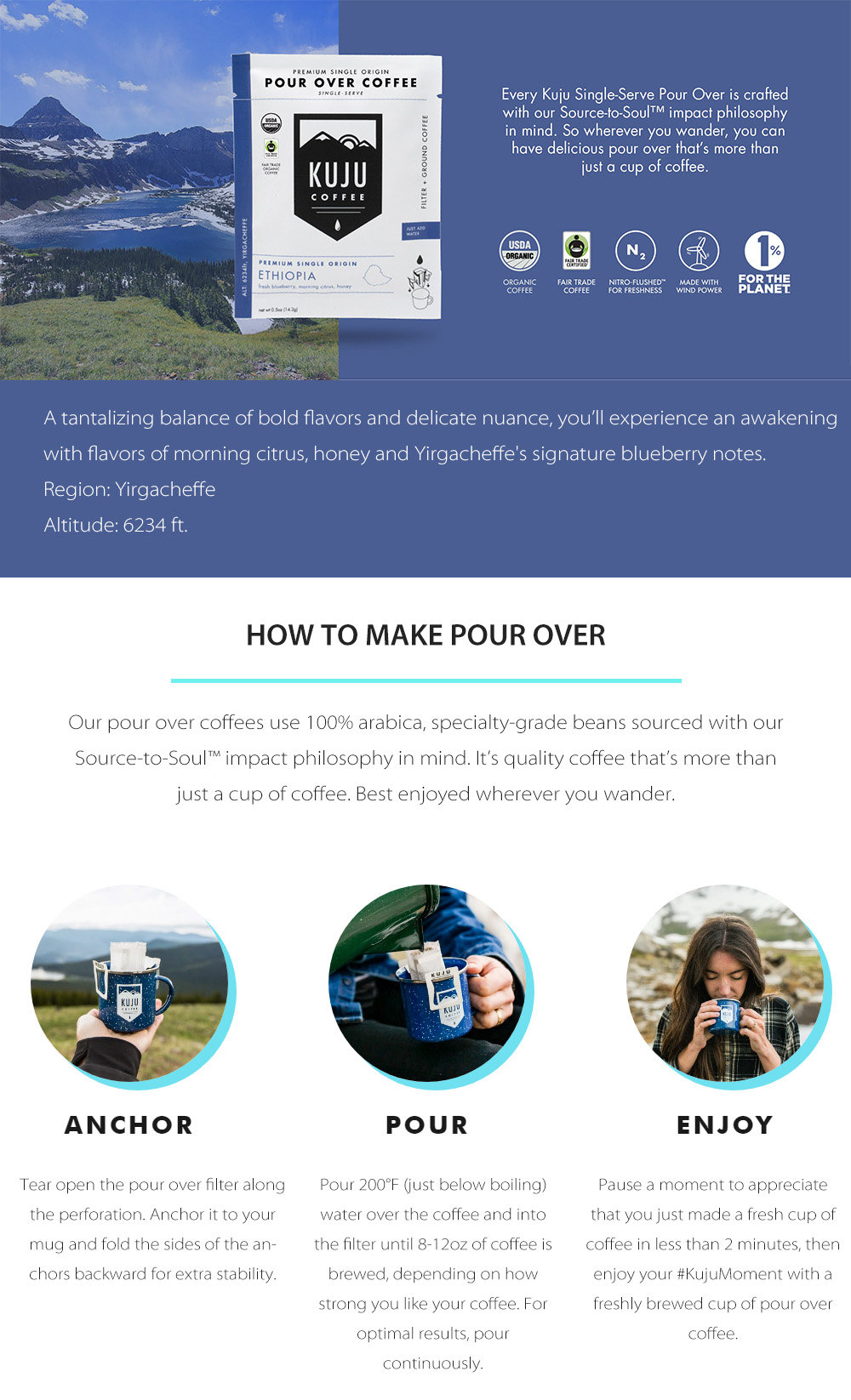The image features a picturesque landscape at the top, showcasing a majestic mountain adorned with lush trees, a shimmering body of water, and verdant grass. Overlaid on this serene backdrop is a prominently placed advertisement for Kuju Coffee's premium single-origin Ethiopia pour-over coffee. The advertisement is styled with a blue-purple color scheme and provides a wealth of information about the product.

In bold text, it highlights the "Source to Soul" philosophy driving Kuju Coffee, ensuring that wherever your travels take you, a delicious cup of pour-over coffee is within reach. The image proudly displays various certifications and commitments, including Organic Coffee, USDA Organic, Fair Trade Coffee, Nitro Flushed for Freshness, Made with Wind Power, and 1% for the Planet, each accompanied by its respective symbol.

Below the main advertisement, text describes the coffee's unique flavor profile: "A tantalizing balance of bold flavors and delicate nuances. Experience an awakening with flavors of morning citrus, honey, and Yirgacheffe’s signature blueberry notes." Additionally, it specifies the coffee's regional origin (Yirgacheffe) and the high-altitude growth conditions (6,234 feet).

The lower section of the image provides a step-by-step guide on how to make a pour-over coffee, illustrated with three small pictures labeled "Anchor," "Pour," and "Enjoy." It instructs users to tear open the pour-over filter, anchor it to their mug for stability, pour hot water over the coffee grounds gradually, and savor the freshly brewed coffee.